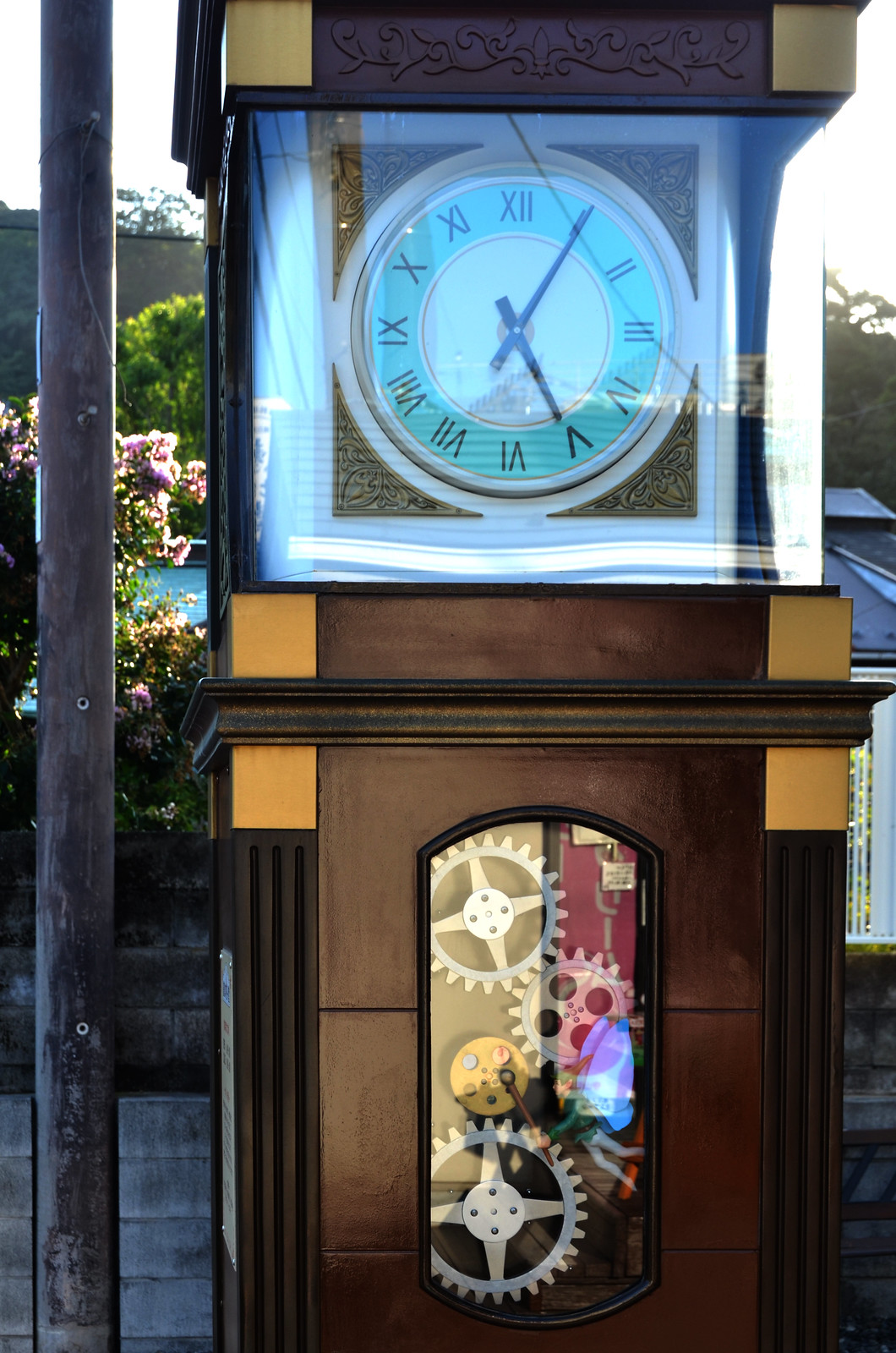This image features a quaint clock tower with a unique design. The central focus is a traditional circular clock encased in a glass box. The clock face is adorned with Roman numerals, which are elegantly displayed on a white and blue band encircling the center. Within this band, the interior is a pristine white circle, showcasing black minute and hour hands that stand out clearly.

Surrounding this circular clock face is a square frame, distinguished by charming yellow fringes that add a touch of classic detail. The entire ensemble is mounted on top of a sturdy wooden box. This wooden base is particularly intriguing, as it includes a small window through which the intricate clockwork gears are visible, offering a glimpse into the mechanical workings of the timepiece.

In the background, lush trees and foliage provide a natural and serene setting that contrasts beautifully with the structured design of the clock tower. The greenery adds depth and context, suggesting that this picturesque clock tower is situated in a tranquil outdoor area.